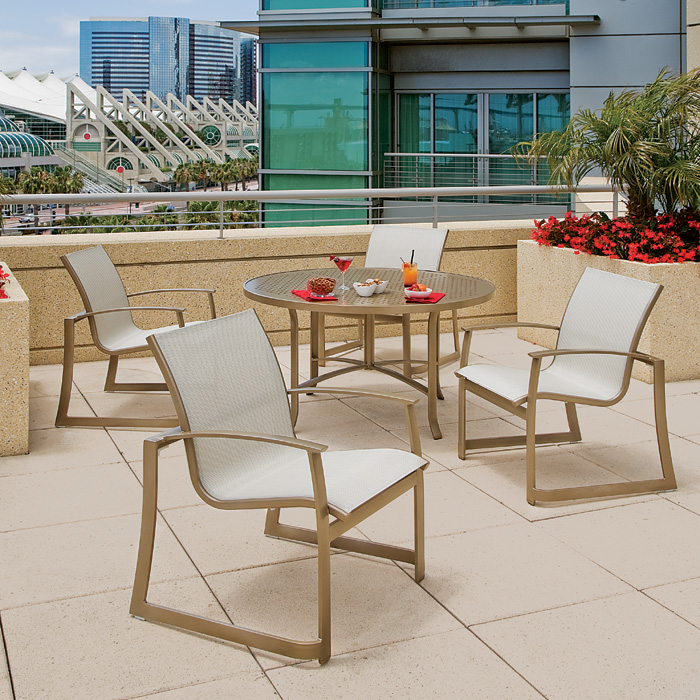This image captures a daytime scene on a rooftop patio, likely in a business or upscale setting. The patio itself is decorated in tan and brown tones featuring a visually striking silver railing. Flanking the patio are planters filled with red flowers and palm-like plants, contributing a bit of natural color to the scene. The focal point is a round, tan table adorned with two red napkins and holding bowls of aperitifs and fruits, along with two cocktails—one red, one orange. Surrounding the table are four stylish chairs featuring white seats and tan armrests. The background reveals an urban vista with multiple business buildings and a walkway lined with palm trees, enhancing the sophisticated ambiance of the rooftop setting.